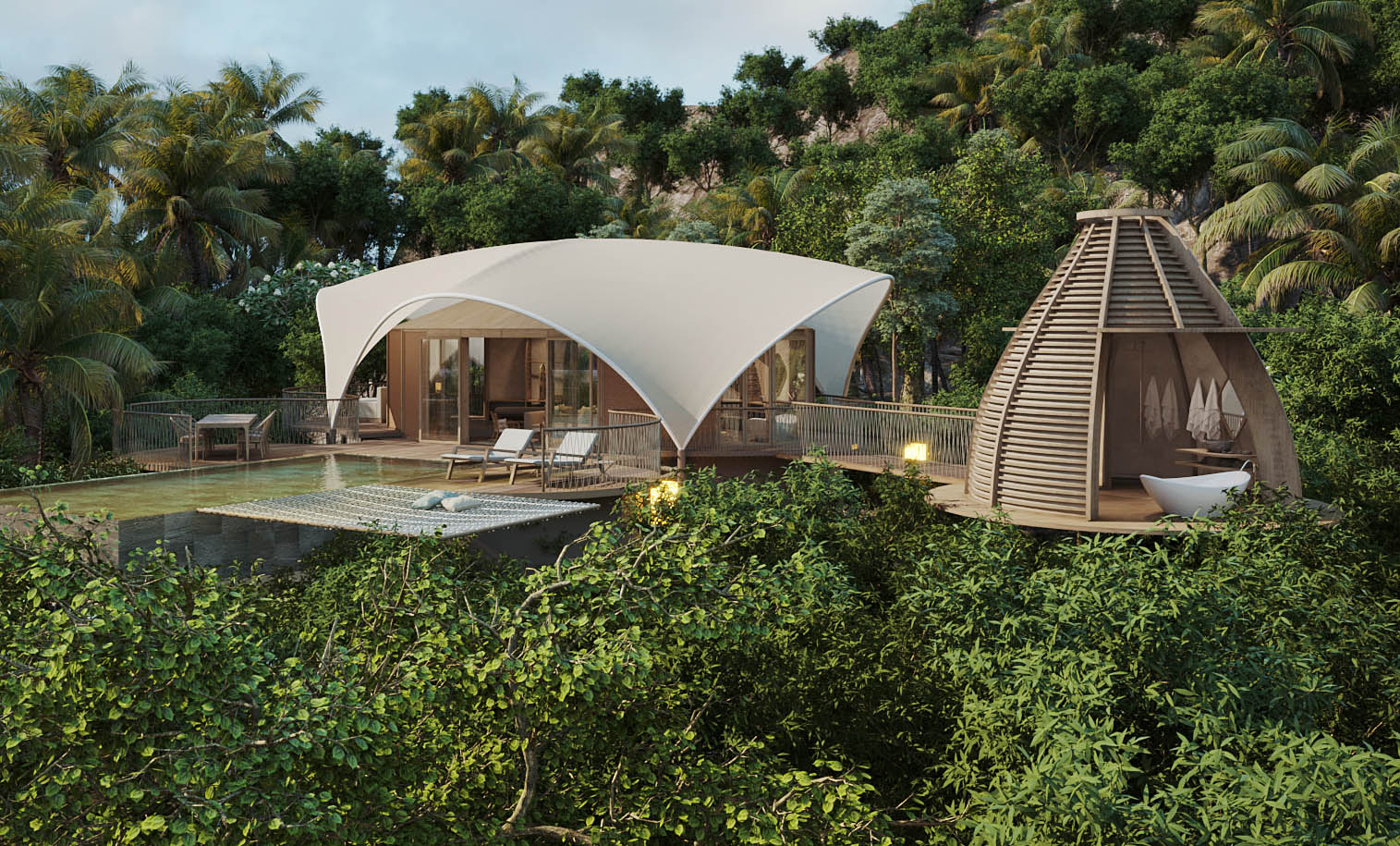The photograph captures an exquisite outdoor setting at a high-end resort or luxurious private estate perched atop a rocky mountain, creating a treehouse-like atmosphere. The central feature is an elevated in-ground pool with marble siding, seamlessly blending with the wooden patio surface. The pool's elevation offers a breathtaking view of vibrant tropical vegetation, including numerous palm trees, cascading down the hillside below.

Adjacent to the pool, an airy gazebo with open sides houses a sumptuous bathtub, allowing visitors to bathe while overlooking the verdant landscape. This gazebo is part of a unique structure that resembles a wooden pod, adding to the charm and exclusivity of the setting. The image also displays another structure adjacent to the pool, which is covered by a white fabric canopy and features a glass-enclosed living area furnished with sofas and chairs, giving it a cozy, inviting feel.

The surroundings provide complete privacy, as the estate is nestled against a hill thick with lush vegetation. Additionally, the property includes a bridge leading to the bathroom area, which is conically shaped and made of wood, with an open window revealing a pristine white bathtub. The blue sky, dotted with white clouds, further enhances the tropical, tranquil ambiance.